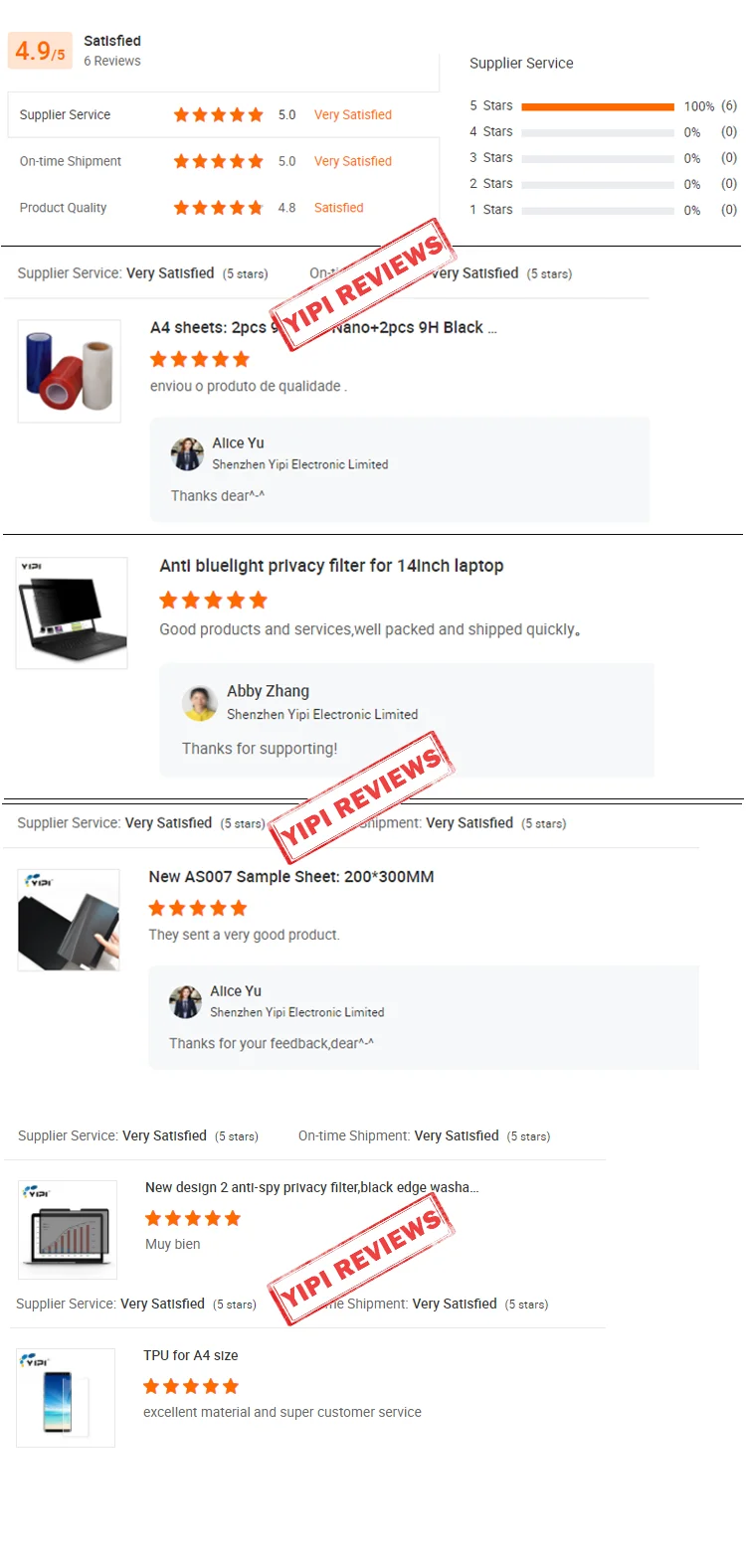This image is a lengthy screenshot likely from a mobile device, featuring a series of product reviews against a white background. At the top, a satisfaction rating of 4.9 out of 5 is highlighted, based on six reviews. The reviews boast perfect five-star ratings in three categories: supplier service, on-time shipment, and product quality, with the stars depicted in orange.

Directly below the ratings, there is a featured product image showing three rolls of colored plastic, labeled as "A4 Sheets, Two Pieces." Over this product entity is a striking red stamp with the uppercase text "YIPI Reviews."

The screenshot continues to present two additional products: an anti-blue light privacy filter and a new "AAS007 Sample Sheet." Both items are marked with five-star ratings and the prominent "YIPI Reviews" stamp.

Extending further, the screenshot includes more reviewed products, revealing a total of two additional items. One of these items features the "YIPI Reviews" stamp placed diagonally across it. The overall length and detail suggest a robust compilation of highly-rated products curated for review.